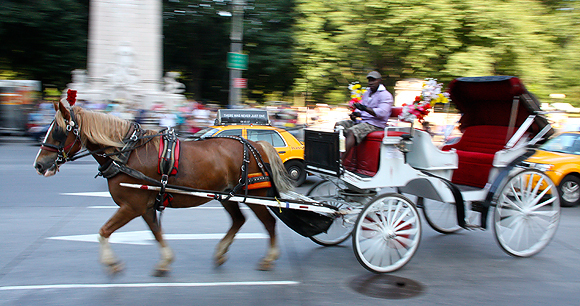A picturesque scene unfolds in bustling New York City, likely near Central Park, featuring a classic horse and carriage amid a vibrant urban setting. The all-white carriage, typical of those seen around Central Park and Columbus Circle, is adorned with velvety red seats and a retractable leather roof, which in this photo is open. A shelf brimming with colorful flowers is positioned just behind the driver's seat. The driver, a black man dressed in a grey baseball hat, a lavender long-sleeve collared shirt, and green shorts, sits at the helm. The sturdy brown horse pulling the carriage is distinguished by a white stripe down its snout and light brown accents on its mane, tail, and hooves. Amidst a fairly busy road, the carriage is flanked by yellow taxi cabs, while a group of people can be seen near a road sign on the opposite side of the street. Towering trees from the park rise towards the top right of the image, adding a touch of natural beauty to this quintessential urban snapshot.